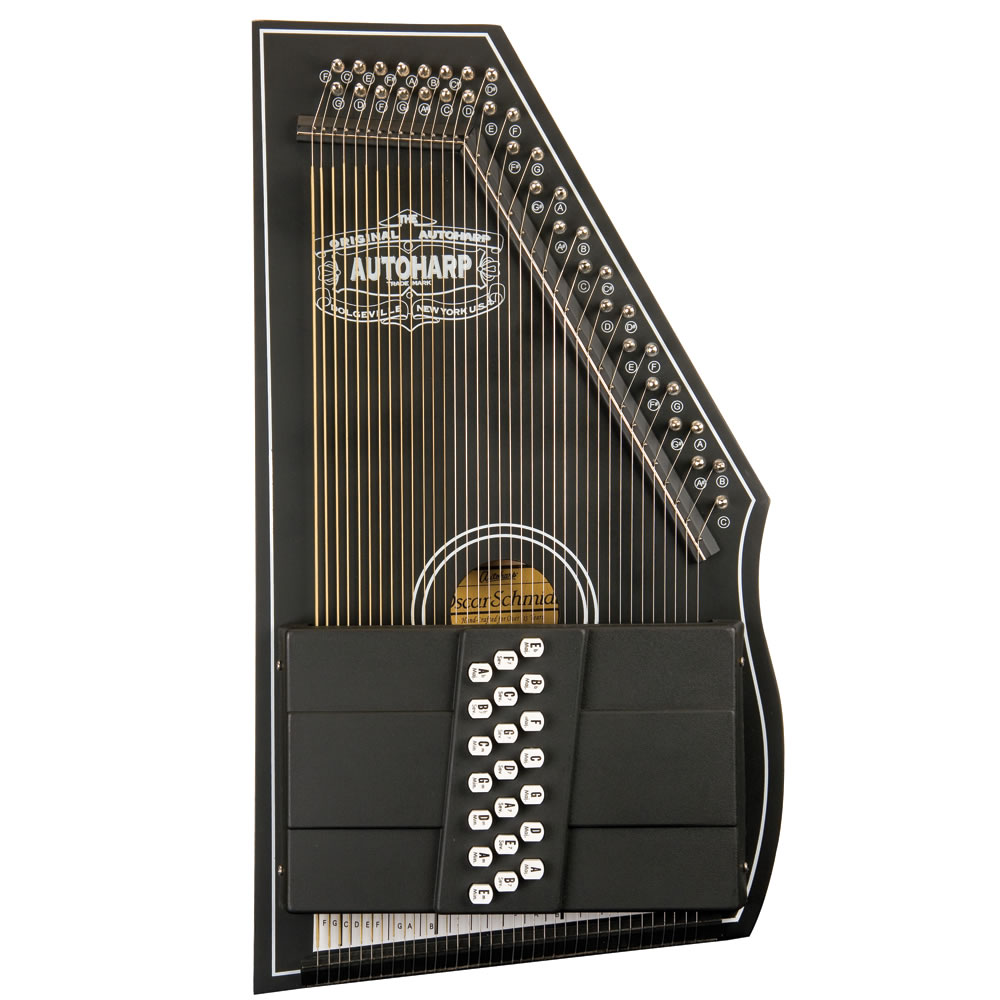This image showcases a strikingly modern and innovative musical instrument known as the autoharp, likely originating from Boulgaville, New York, USA. The instrument is predominantly black with a contrasting white pinstripe outlining its perimeter. The design features a straight vertical left side that turns sharply at the top, creating a steep angle that transitions into a very shallow S-shape on the right before angling back towards the left at the bottom. 

The autoharp has around 50 golden-colored strings, each equipped with tuning knobs positioned on the top. Adjacent to each tuning knob is a small circle marked with a white number or letter. The middle section of the autoharp integrates a keyboard-like panel with white buttons inscribed with black letters, oriented 90 degrees to the right.

Notably, the instrument prominently displays "Original Autoharp" in white text beneath the strings, along with a gold emblem featuring a white circle at the bottom. The eye-catching "Messo" logo is also visible in bold white text amidst the predominantly black instrument body. The autoharp's sophisticated appearance suggests that it is likely an expensive piece, reflecting high craftsmanship and a modern twist on traditional design.